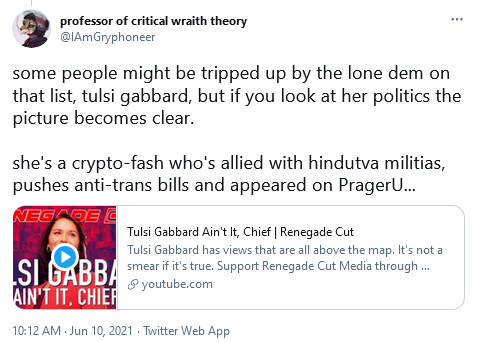The image depicts a Twitter page belonging to the user "Professor of Critical Wraith Theory," whose handle is "@IAmGriffin." The profile photo showcases an anthropomorphic animal wearing a hoodie. A tweet from June 10th, 2021 at 10:12 a.m. is prominently displayed. 

In the tweet, the user comments on Tulsi Gabbard, an American politician, noting that she is a "crypto-fascist" with affiliations to Hindu militias, proponents of anti-trans legislation, and has appearances on the right-leaning educational platform PragerU. The tweet is accompanied by a screen-capture from PragerU and a pinned YouTube video titled "Tulsi Gabbard Ain't It - Chief Renegade Cuts." The user also encourages supporters to follow Renegade Cup Media and concludes with the statement, "Tulsi Gabbard has views that are all over the map. It's not a smear if it's true." The post is in black font on a white background, making the text stand out clearly.